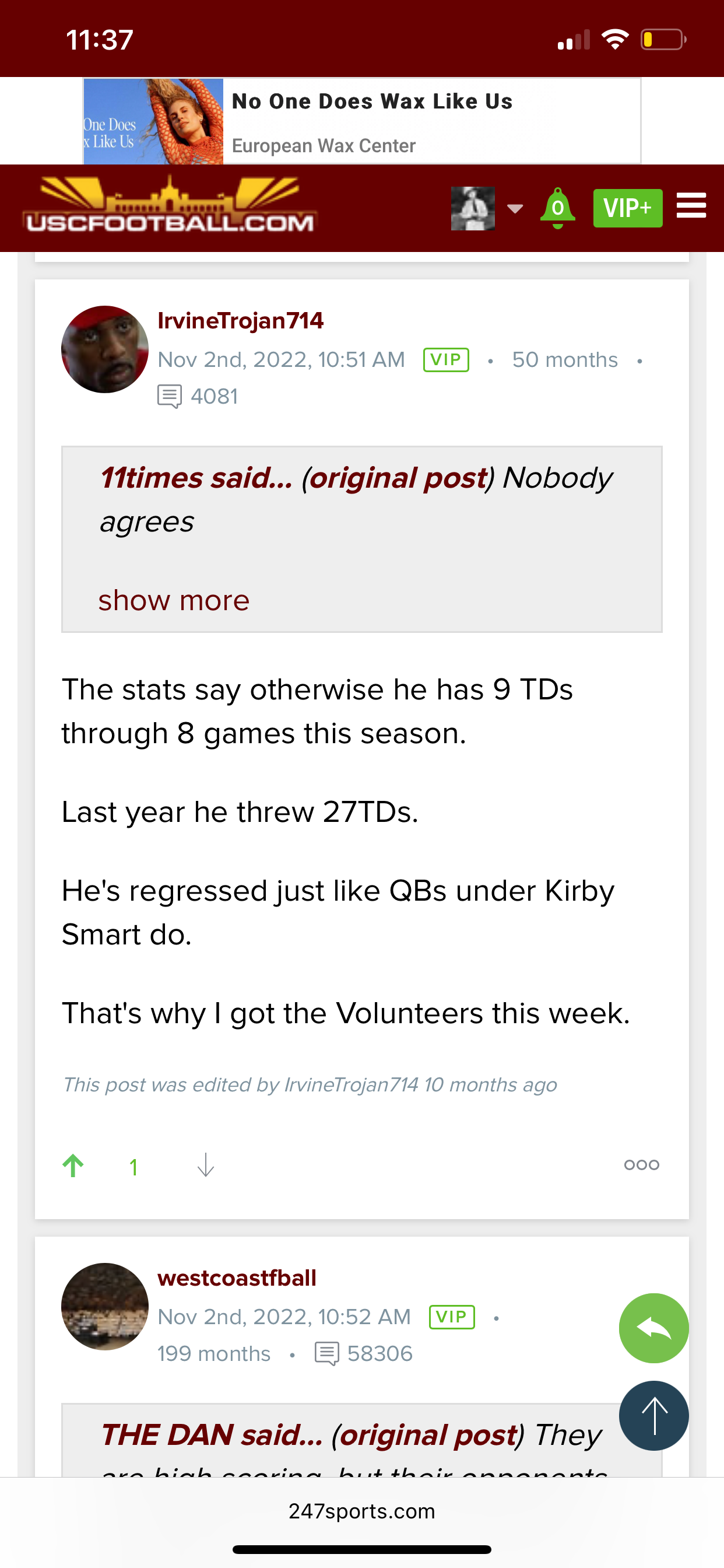**Category: Websites**

The image captures a phone screen with notable details:

- **Time and Status:** The top maroon bar of the screen displays the time at 11:37. It's unclear whether it's AM or PM. The Wi-Fi is enabled, but the battery is indicated as almost dead. 
- **Advertisement:** Beneath this bar, there is a white space with the text "No one does wax like us. European Wax Center." This section includes an image of a person jumping with both arms up against a blue sky background, wearing orange.
- **Website Interface:** Below the advertisement, another maroon bar is visible with the text "uscfootball.com." This bar includes a notifications button, a VIP Plus button, and a menu button. 
- **User Profile and Post:** The screen also shows a user profile belonging to "Irvine Trojan 714," with a profile picture. The post is dated November 2nd, 2022, at 10:51 AM, and the user is identified as a VIP member for 50 months. 
- **Post Content:** The post states, "11 times said, nobody agrees. Show more. The stats say otherwise; he has 9 TDs through 8 games this season. Last year, he threw 27 TDs. He has regressed just like QBs under Kirby Smart do."

The overall presentation denotes a mixture of a mobile web page display with promotional content and a football-related user discussion, emphasizing comprehensive statistics and user interaction features.